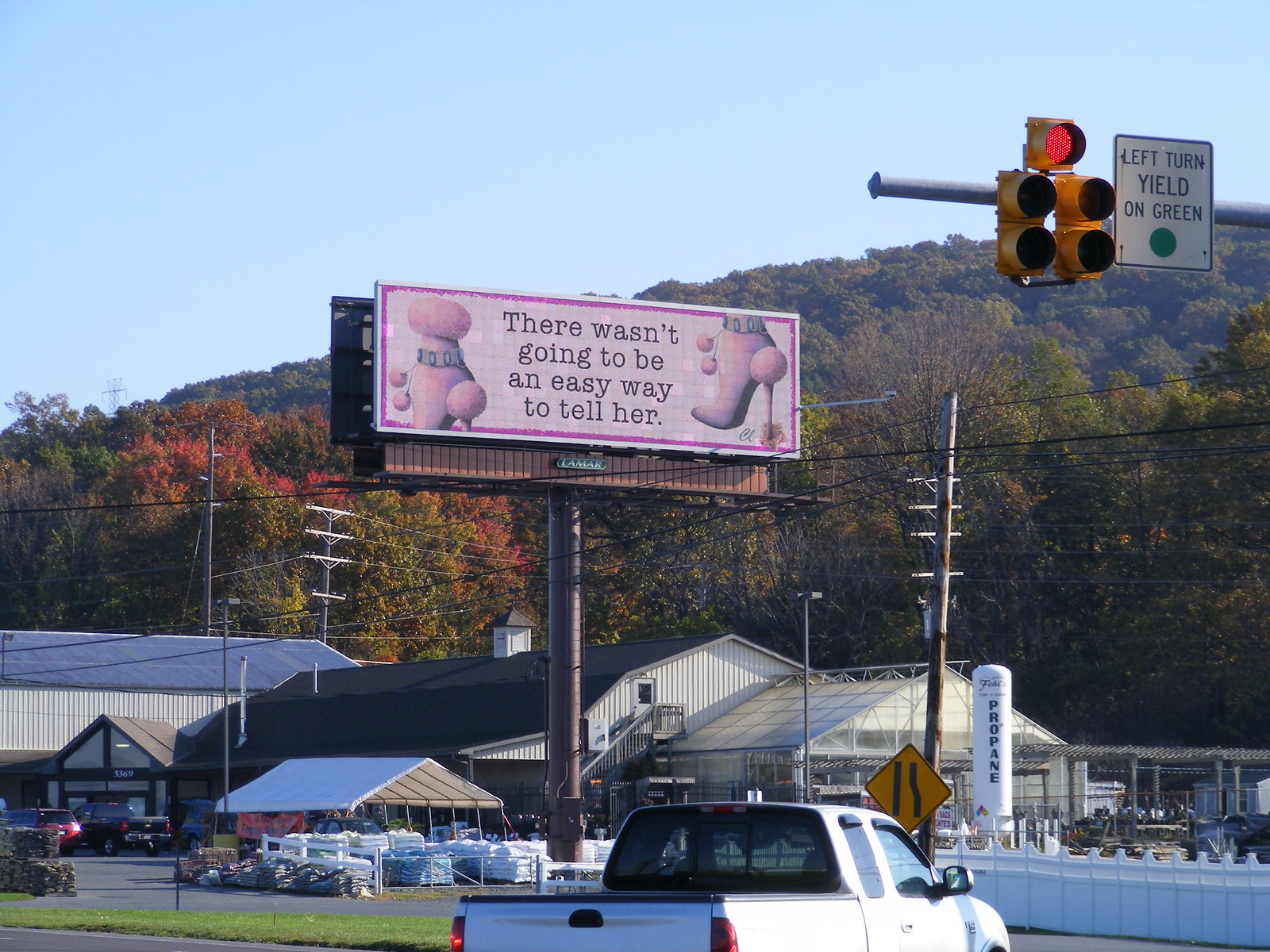In this outdoor photograph, a farm store forms the backdrop, characterized by its gray exterior and black roof. A notable feature of the scene is a prominent pink billboard located in front of the store, bearing the intriguing message, "There wasn't going to be an easy way to tell her." The store is set against a busy parking lot that lies just across the road, where a white pickup truck is parked prominently in the bottom middle of the image. The truck is surrounded by large bags, which likely contain either mulch, fertilizer, or dirt, stored under makeshift tents. A substantial white tank labeled "propane" is also visible, contributing to the rural and industrial feel of the setting. Additionally, a sturdy white fence runs horizontally in front of the truck and the store, adding a touch of order and structure to the bustling environment. The building also features an exterior staircase leading to a door on the top floor, hinting at a functional, utilitarian design.